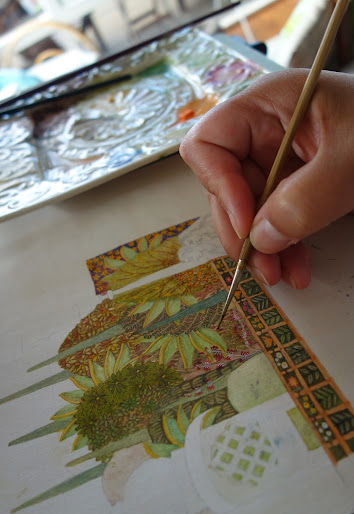In this well-lit indoor photograph, we observe a close-up of a hand with tan skin delicately holding a slender paintbrush. The individual appears to be right-handed, but their gender is indeterminate from the image. They are engrossed in creating a highly detailed and unfinished painting depicting flowers and intricate designs with earthy tones, including shades of green, gold, and brown.

The painting-in-progress is being executed on a flat surface, likely an art table, where the artist is currently applying paint just below a flower. To the right of the painter's hand lies a silver tray with a few stray paint drops, perhaps where the artist disposes of excess paint. Additionally, there is a white, slightly blurry square plate in the background, adorned with floral embroidery and various paint splotches, including orange, blue, and pink. This plate, which also holds a couple of thicker paintbrushes, appears to serve as the palette for mixing or cleaning the paintbrush.